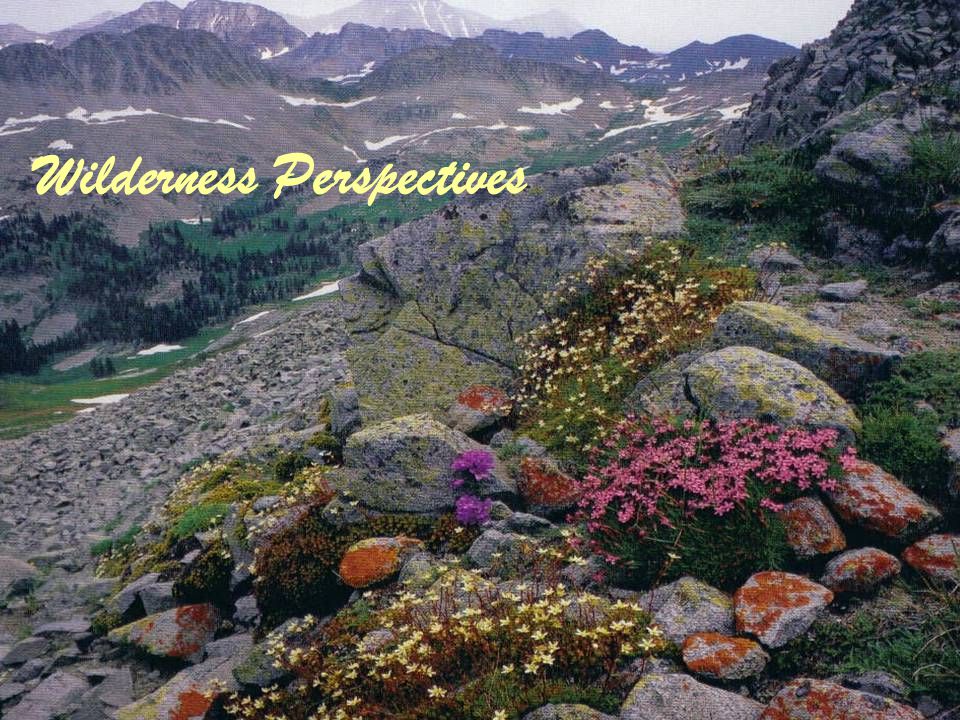The image is a low-quality color photograph with a granular texture, possibly due to being printed on textured paper or scanned. It features a stunning mountainous landscape in landscape orientation. In the foreground, the photograph displays a variety of multicolored wildflowers growing among moss-covered gray and black porous rocks. Some of these rocks have a rust-colored moss on them. The wildflowers are small and clustered, with hues of white and pink. 

Below the wildflowers, there is a mix of grass and stones. The landscape slopes from the center of the image downward to the left, leading the eye to a lush green valley with patches of snow. The valley is fringed by stands of dark green trees, which rise up against distant, snow-capped mountain ranges. The overall scene appears to be taken in the middle of the day. 

At the top left of the image, there is brush-style cursive text in a cream-yellow color reading, "Wilderness Perspectives," adding an artistic touch to this representational realism photograph. There is no additional text or border framing the picture, emphasizing its natural beauty.